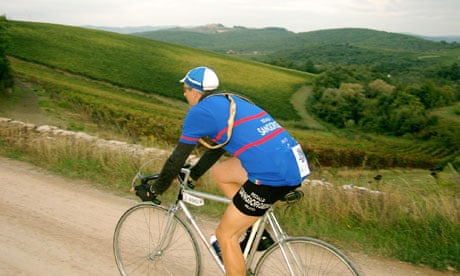The image captures a lone cyclist navigating a well-worn, light sandy tan dirt trail amidst a scenic countryside landscape. The cyclist, adorned in black biking shorts, black sleeves, and gloves, sports a blue and red striped jersey over a long-sleeved black shirt. A distinctive blue and white cap, styled like a beanie, tops his head for protection. He rides a sleek, silver-colored bike along the stone-lined path. The background is a vibrant tapestry of gently sloping green hills, dotted with clumps of bushes, some trees, and patches of wheatgrass, under a cloudy sky with hints of sunlight breaking through. A three-foot stone wall with uniform green weeds growing around it adds rustic charm to the serene, almost solitary setting, emphasizing the cyclist's focused journey on the dirt trail.